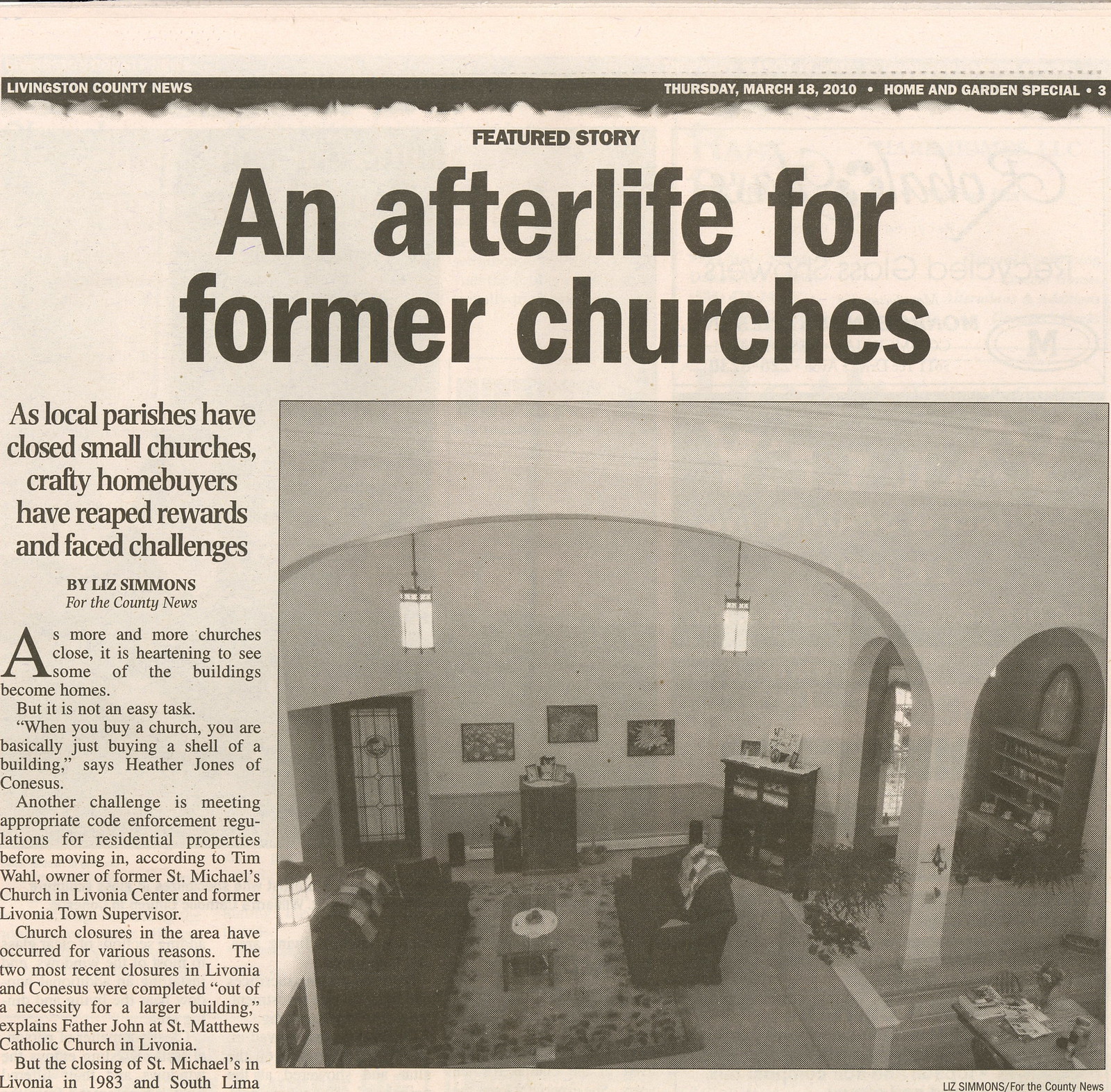The image is a black and white photograph from a newspaper article titled "An Afterlife for Former Churches," published in the Livingston County News on Thursday, March 18, 2010, as part of their Home and Garden Special. The featured story by Liz Simmons explores the trend of converting closed church buildings into residential homes, highlighting the rewards and challenges faced by homebuyers. The photo captures the front lobby of a repurposed church, now a residential space. The setting is indoors, showing high arched ceilings adorned with two hanging lights, creating a charming and welcoming atmosphere. The room is furnished with a loveseat, a carpet, a credenza, a coffee table, and paintings on the wall. A door and a bookcase are visible in the right-hand corner, and what appears to be a desk is partially seen in the bottom right-hand corner. The accompanying text quotes various local figures discussing the complexities and satisfactions associated with such transformations, emphasizing that while buying a former church provides a unique opportunity for homeowners, it comes with the need to meet specific residential code requirements. The readership is informed about recent church closures in Livonia and Cornasis, noting both practical and historical aspects.